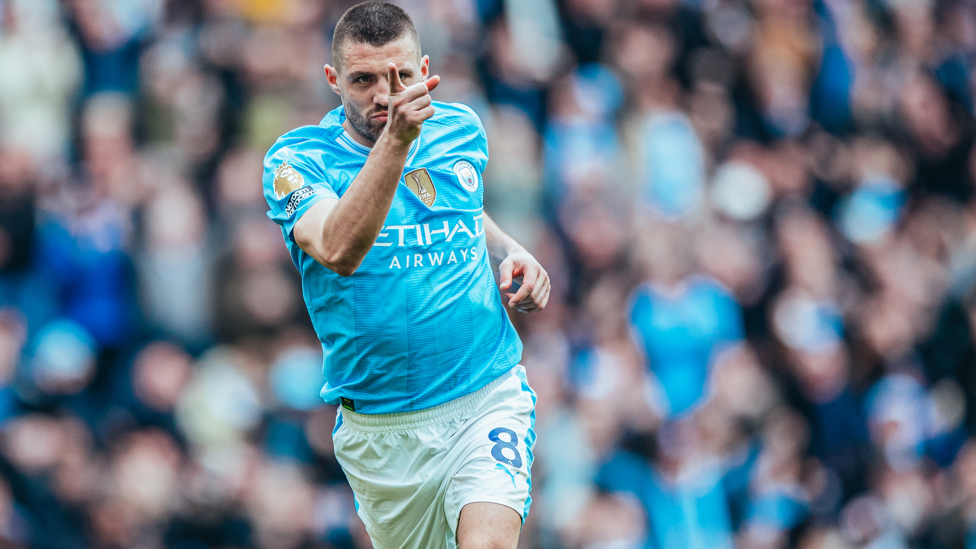The image is a high-quality color photograph of a male professional soccer player, widely known as a football player in Europe. He is positioned in the middle of a soccer match, running and pointing forward with his right hand, with the index finger slightly raised. The player has short, dark grey hair, a beard, and a mustache. He is wearing a blue jersey emblazoned with the white text "ETIHAD Airways," confirming the sponsor, and is part of the Manchester team, as indicated by the FIFA patch and the visible lettering on the jersey. His uniform also includes white shorts, marked with the number 8 in blue on the left leg. The player's expression is one of excitement, possibly celebrating an achievement. The background depicts blurred faces of cheering fans, donned in white and blue attire. The athlete's pose, combined with his intense focus and the vibrant atmosphere, captures the dynamic and thrilling nature of the game.